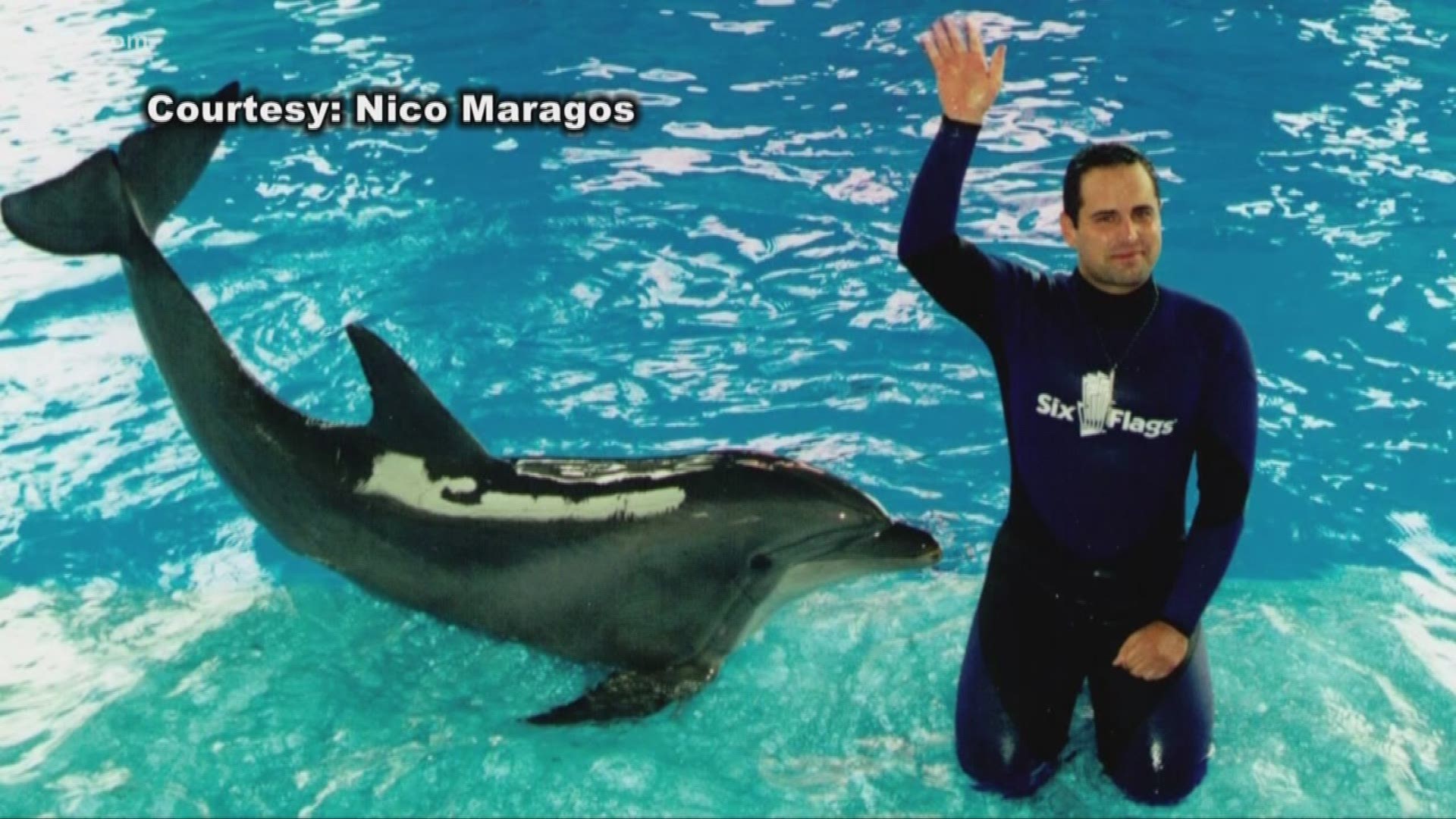This captivating photograph serves as an advertisement for Six Flags, capturing a moment between a young dolphin trainer and a playful dolphin. The trainer, a young white man with short dark hair, is wearing a black full-bodied wetsuit adorned with the Six Flags logo and white lettering. He has a whistle around his neck and is kneeling on a shallow water shelf in front of a deeper, strikingly vivid blue pool. His left hand rests on his thigh while his right hand waves enthusiastically at the camera. Beside him, the dolphin is positioned on its stomach with its tail raised high in the air, as if mimicking the trainer's wave. The dolphin’s nose points towards the trainer, emphasizing their close bond. The text in the upper left corner of the image reads "Courtesy Niko Maragos," adding a personal touch to this joyful and engaging scene.